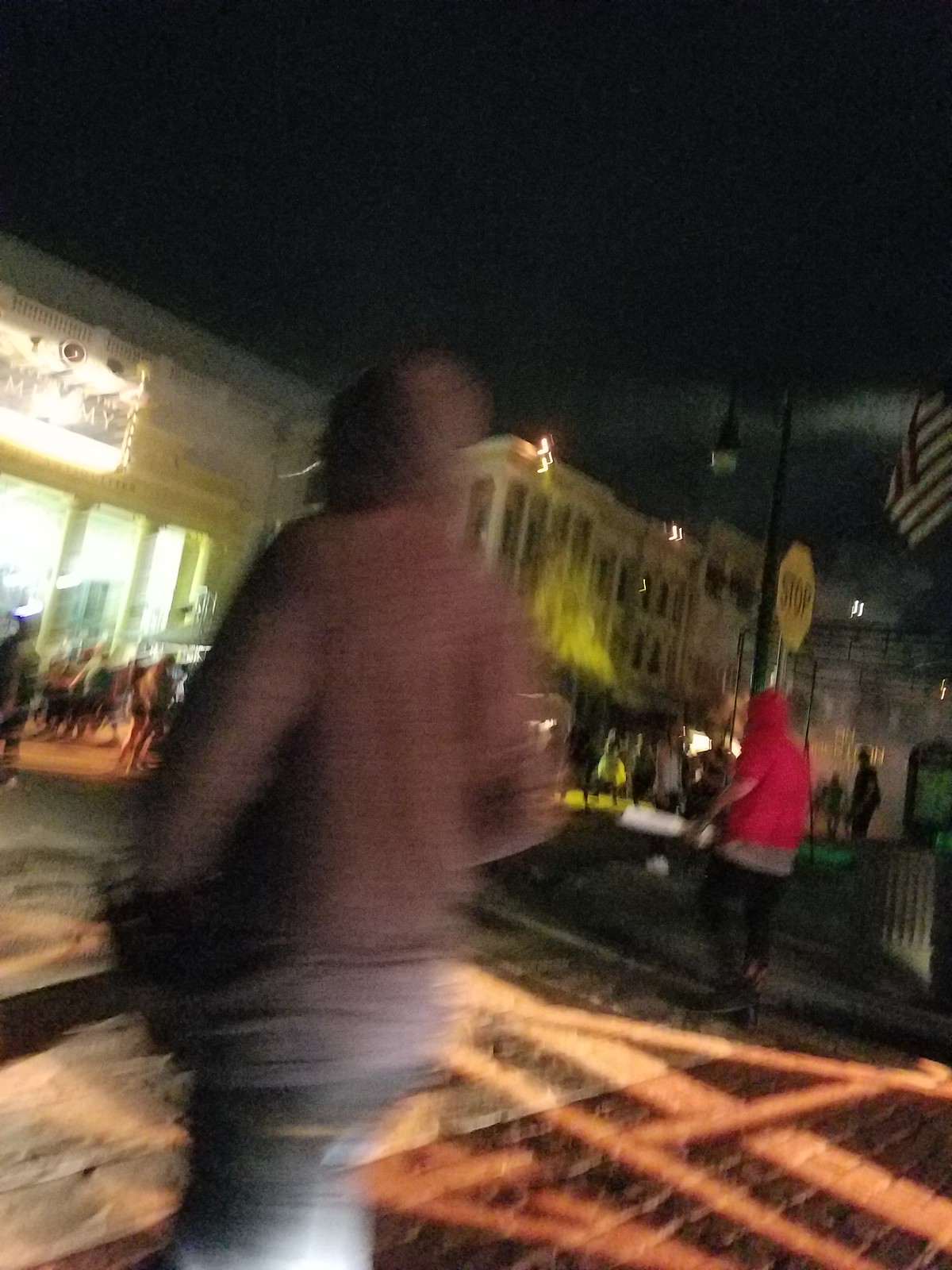In this blurry city photo, the main subject in the foreground is wearing a maroon hoodie pulled over their head, with a gray shirt peeking out from underneath and blue jeans. They appear to be crossing a street on a crosswalk heading towards a store. The store features a lit-up sign, large windows that extend from approximately 10-12 feet high to the ground, and is supported by white pillars. The sidewalk is bustling with many people walking and entering or exiting the store. To the right of the main subject, another person in a short-sleeved red hoodie, also wearing a gray shirt underneath and black pants, is also crossing the street. In the background, there are taller city buildings characterized by their white façades and pillars extending several stories high. Behind the person in the red hoodie, a street lamp is visible with a stop sign attached to its pole. The upper right corner of the image features a partial view of an American flag against a dark, cloud-speckled sky.